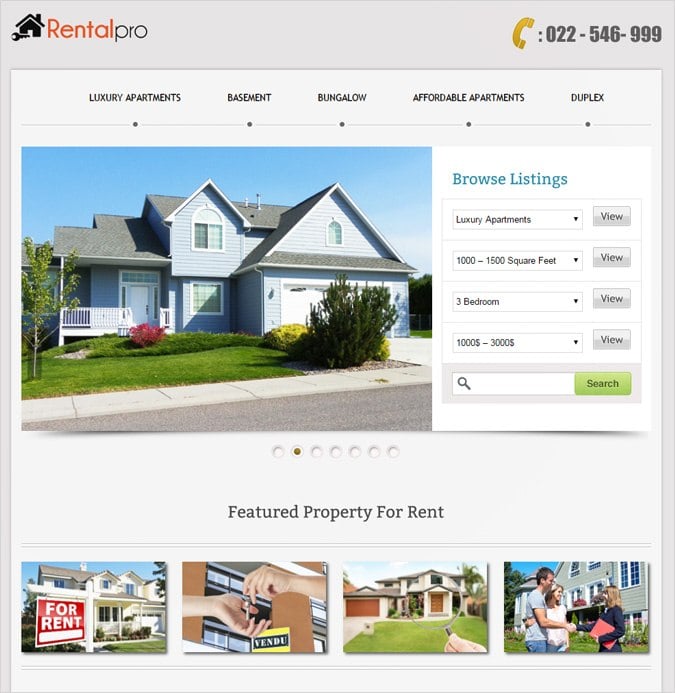The image depicts a website dedicated to property rentals. At the top, a grey banner stretches across the page, prominently featuring a cartoon or clipart image of a house coupled with a key. Beside this image, the text "Rental Pro" is displayed, with "Rental" in bold red font and "Pro" in standard black font.  

To the right within the same banner, there is a golden-yellow telephone icon accompanied by a phone number in grey font, providing a contact option for potential renters.  

Beneath this header is a navigation bar with categories such as "Luxury Apartments," "Basement," "Bungalow," "Affordable Apartments," and "Duplex," enabling users to easily navigate to their preferred type of rental property.  

The main section of the page showcases a large image of a house. This property features a grey roof, a blue wooden facade, a white wooden porch, and white trim around the windows. The house also includes a white garage, a neatly maintained front yard with grass and shrubs, and a visible pavement and road in the foreground.  

To the right of the house image, the text "Browse Listings" appears in blue font, followed by search parameters that include filters for "Luxury Apartments," desired size, number of bedrooms, and price range. Below these filters, a search bar is available for users to input custom criteria. Additionally, there are several thumbnail images that users can click to view more pictures of the house.  

Further down, the words "Featured Property for Rent" introduce a section with four generic images. These images include a house labeled "For Rent," a set of keys being handed over, a house with a magnifying glass highlighting it, and a couple either receiving keys or shaking hands with a real estate agent in front of a house.